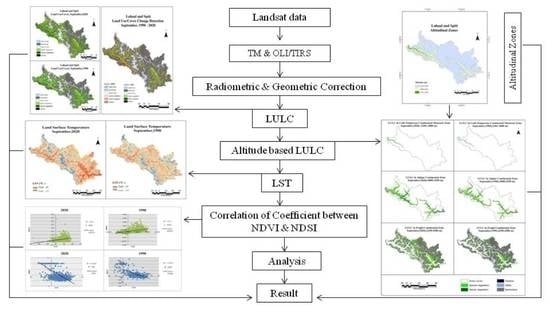The image is a detailed infographic in landscape orientation, presenting a structured flowchart for topographical analysis. Central to the flowchart, a series of rectangular boxes with black-trimmed borders are aligned vertically and connected by arrows, guiding the reader through the sequential steps of data processing and analysis. 

Starting at the top, the boxes are labeled as follows: 
1. Landsat Data 
2. TM and OLI/TIRS 
3. Radiometric and Geometric Correction 
4. LULC (Land Use and Land Cover)
5. Altitude-Based LULC
6. LST (Land Surface Temperature)
7. Correlation of Coefficient between NDVI (Normalized Difference Vegetation Index) and NDSI (Normalized Difference Snow Index)
8. Analysis 
9. Result

Flanking this central column, there are sixteen sub-charts—nine on the left and seven on the right—that correspond to various states and overlays of the landmass, rendered in blues, greens, and oranges. These sub-charts illustrate specific land properties and measurements, visually supporting the data described in the central flowchart. The entire visual aids in understanding the interrelated processes of topographical and geographical analysis, from data acquisition through final results.